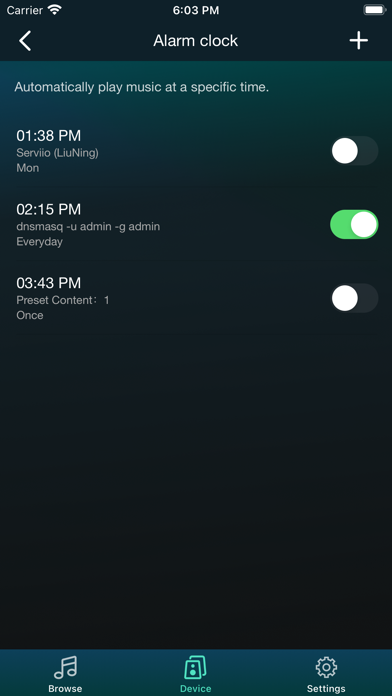A digital alarm clock interface is prominently displayed at the top of the screen, showcasing a battery status icon indicating a nearly full charge. To the left, the screen shows the word "carrier," with no specific brand mentioned, accompanied by a Wi-Fi logo on the right. Centrally aligned is the text "Alarm Clock" with the current time displayed above it. To the left of the "Alarm Clock" title, there's a left arrow button, and to the right, an option to add an alarm.

The display transitions from a lighter black at the top to a darker black towards the bottom. Just below the central text, a box with the option "Automatically play music at a specific time" is visible. Beneath this box, at 1:38 PM, the name "Servio Liu" is mentioned, followed by "mine" and slider buttons indicating various settings. At 2:15 PM, additional administrative settings are displayed with an indication that these settings are activated, as shown by the green slider button.

At 3:43 PM, preset content one is identified with a slider button set to the left, meaning it is not active. The bottom of the screen features a blue navigation bar with three options: "Browse" (indicated by a music note), "Device" (highlighted in green and indicated by two speakers), and "Settings" (represented by a gear icon). The device option is currently highlighted in green, signifying its active status.